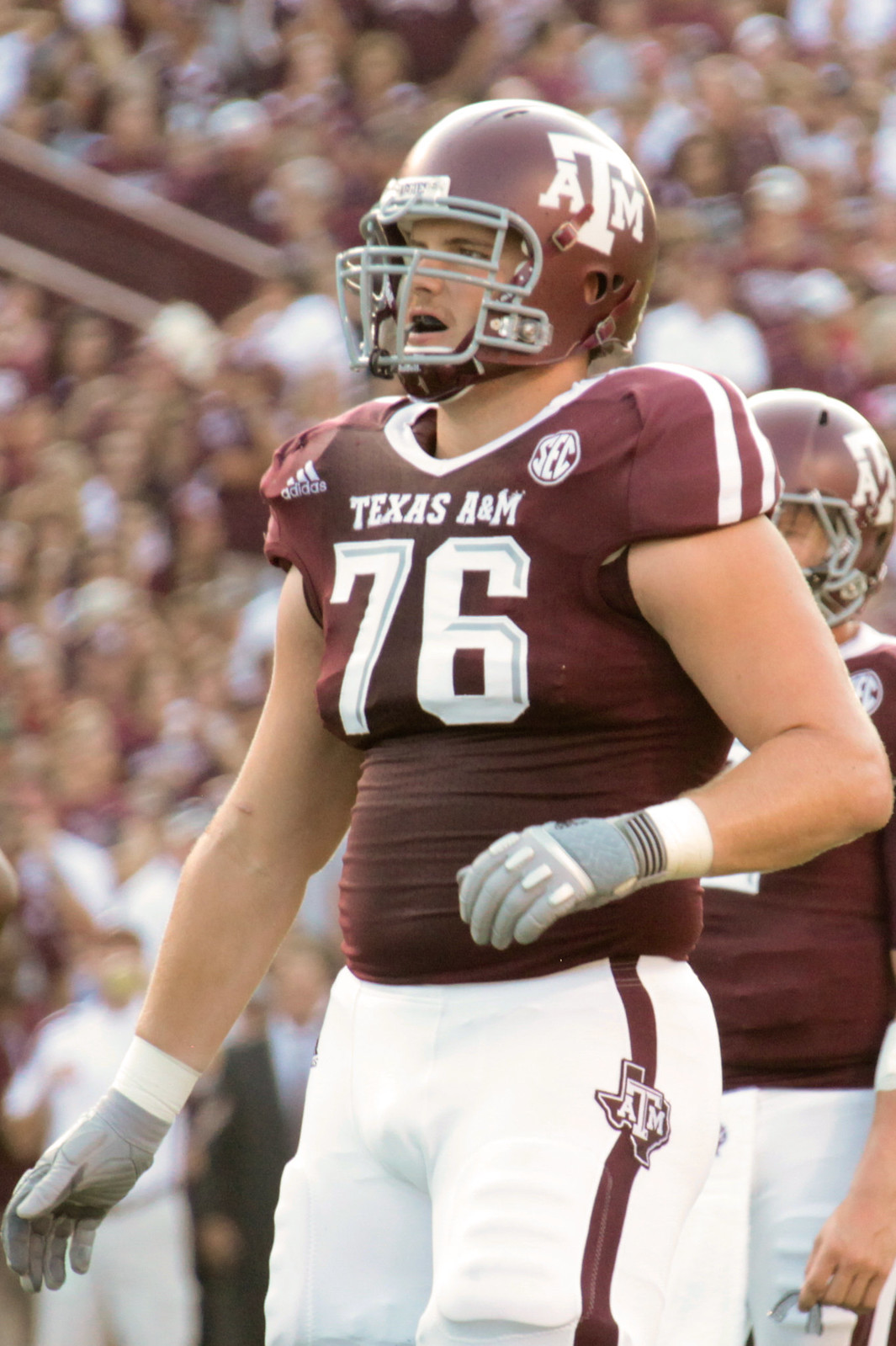This detailed photograph, taken outdoors during a daytime football game, captures an American football player from the Texas A&M team, positioned centrally in the image and facing slightly to the left. The player is wearing a maroon short-sleeve jersey with the number 76 in white letters and a matching maroon helmet adorned with the letters ATM. His uniform includes an Adidas logo on one shoulder and a SEC logo on the other. The player's white pants feature the ATM logo inside a silhouette of Texas running down the leg. He wears gray and white gloves, with his left arm bent at the elbow and his right arm extended forward. His facial expression suggests shock or surprise, with his mouth open. Behind him, another player in the same uniform is partially visible. The background is blurred, showing a crowd of fans in stadium seating, drawing all focus to the player in the foreground. The photo is in portrait mode, capturing the scene from about mid-thigh up.